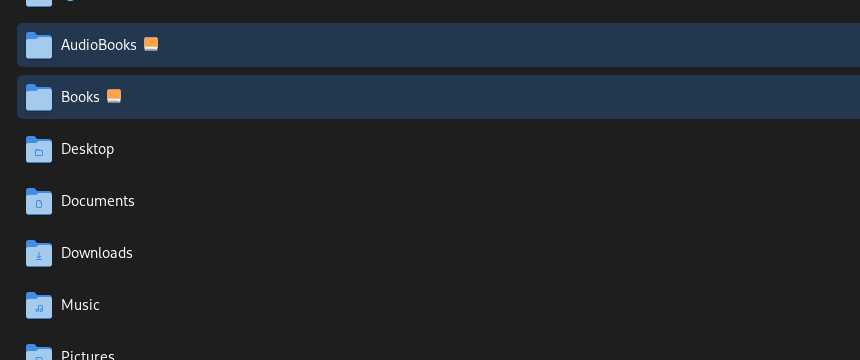The image depicts a computer screen capture with a clear resolution, featuring a black background. The screen displays a file explorer with a column of folder icons and text labels. The text is primarily in a pale blue font with some white elements. 

On the left side of the image, there is a vertical list of folder icons and labels. Each item has a blue folder icon except for the first two, which feature an orange square instead. The labels, in order, are "Audiobooks" and "Books," each highlighted with a navy blue bar, indicating they are selected. Following them, without the highlighting, are "Desktop," "Documents," "Downloads," "Music," and "Pictures."

Towards the top of the image, there's a partial view of an additional folder, but the text label for this folder is cut off and unreadable. The image is clear, and there is nothing else of notable mention in the screenshot.